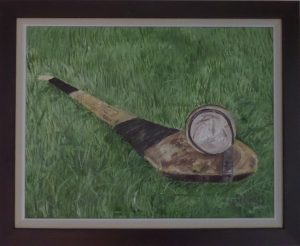The image depicts a detailed painting or drawing of a cricket bat lying on a bed of long green grass. The wooden bat, which has a rounded and flattened end, features two sections wrapped in black tape—one near the handle and the other closer to the base. Resting on the wider end of the bat is a white ball with black stitching, resembling a baseball but with black instead of the traditional red. The image is set within a white mat and framed with a black border, suggesting it is displayed on a wall.